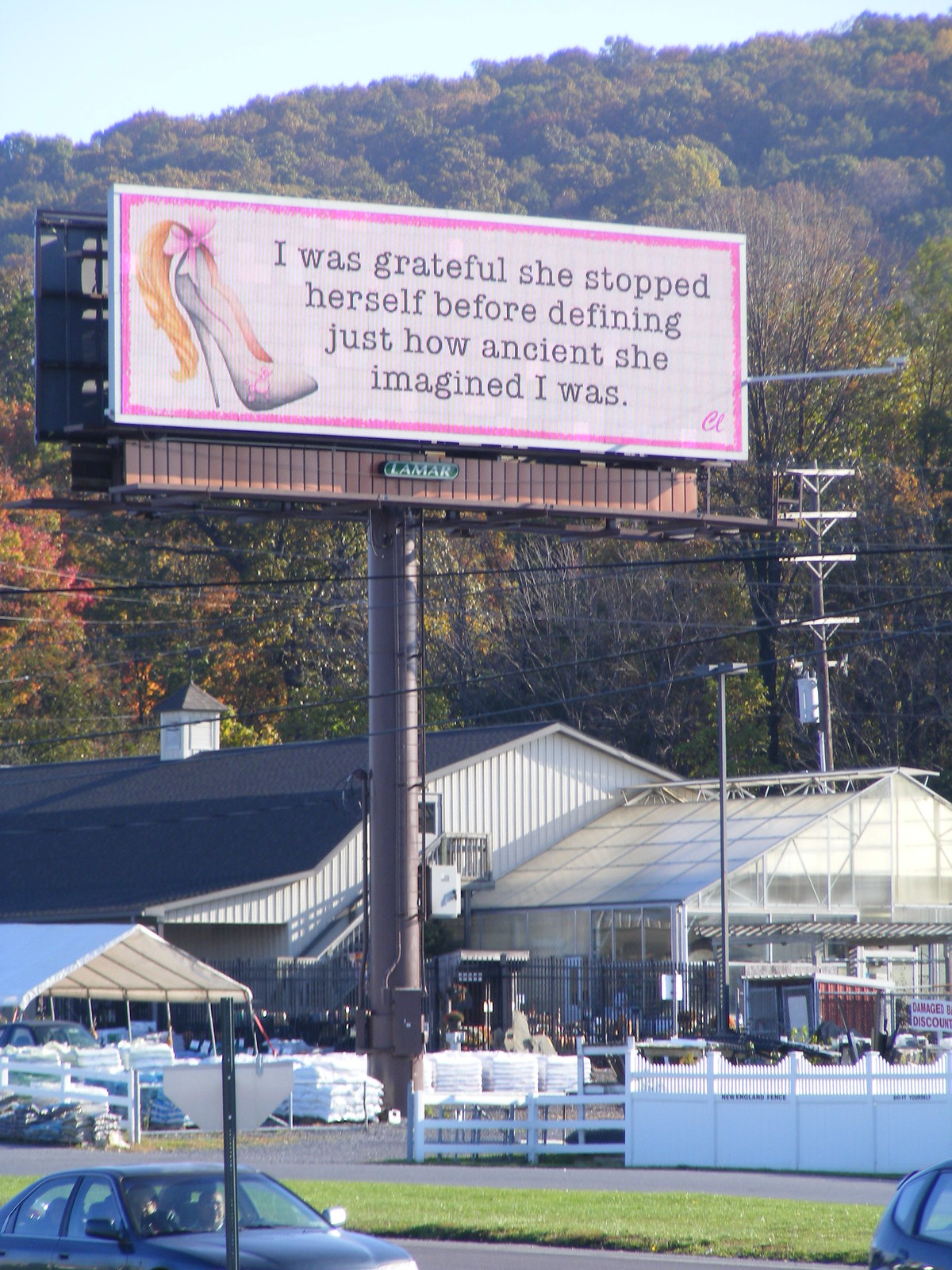This vibrant color photograph captures a bustling roadside scene dominated by a large, eye-catching sign. At the forefront of the image, a sprawling green lawn stretches out, just barely encroached upon by the tops of several parked cars. Just behind this foreground are various buildings, some notably featuring modern glass roofs, standing in stark contrast to the natural elements around them. A lively crowd of people gathers in front of these structures, their presence adding a layer of excitement to the scene. A low wall separates the people from the area behind them.

Further back, the scenery transitions into a lush forest area teeming with green trees, some of which are already sporting a fall palette of golden orange leaves. These trees extend up a gentle hill that fades into the distance. Above, the sky is a clear, serene blue, providing a picturesque backdrop for the landscape.

The centerpiece of the photograph is a large, rectangular sign standing proudly beside the road. The sign features a pink border surrounding a pale pink interior, immediately drawing the viewer's attention. On the left side of the sign, an illustration of a stiletto shoe adorned with a whimsical yellow and pink feather stands out. To the right, bold black text reads, "I was grateful she stopped herself before defining just how ancient she imagined I was." The sign's playful design and mysterious message add a touch of intrigue and humor to the overall scene.